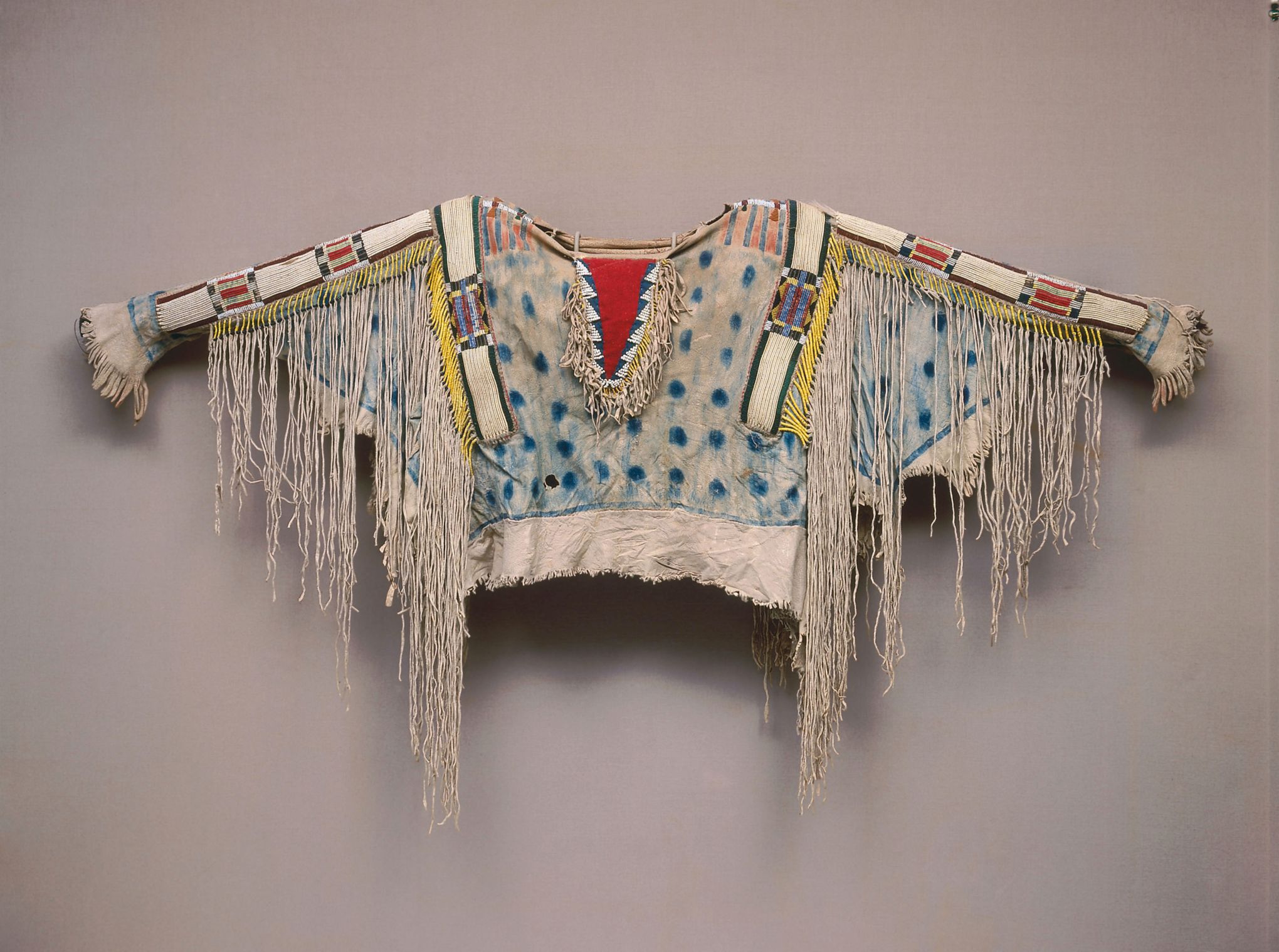Displayed on a white wall, the image features a color photograph of a distinctive shirt that appears to be inspired by indigenous American design. The body of the shirt is crafted from a white fabric adorned with blue polka dots. The shirt has a cut-off style with spread-out sleeves, which are beautifully embellished with stripes of beaded fabric in alternating white and red hues. These decorative elements extend down the arms as canvas-like belts, ending in long white tassels and fringes. The shoulders and sleeves are further adorned with natural-colored, waist-length fringes that add an intricate texture. The shirt also features a v-neck, bordered with a pattern of white and blue beads, and reveals an interior lined with red material, enhancing its vibrant and eclectic aesthetic.